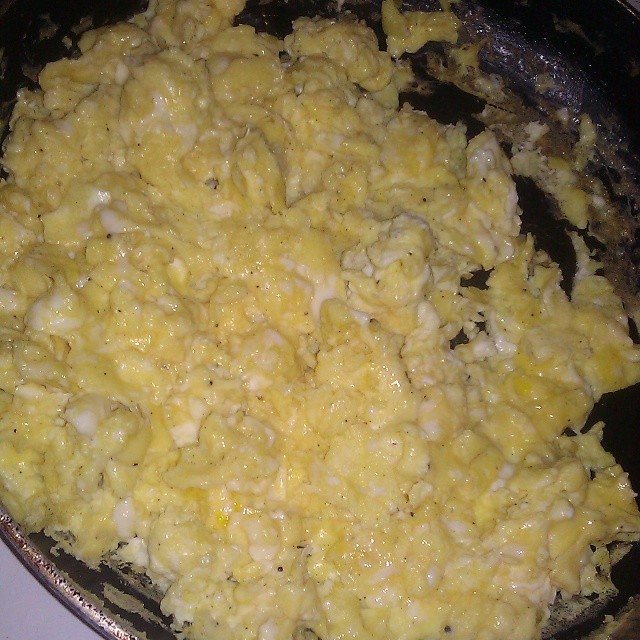This photograph showcases a detailed close-up of a homemade skillet meal, primarily featuring freshly cooked scrambled eggs. The eggs, a mixture of yellow and white, are speckled with pepper and appear shiny, possibly due to being slightly wet or glossy from the camera's flash. The image is tightly cropped, emphasizing the food with only a small portion of the distressed, well-worn skillet visible in the lower left corner, revealing its surface is peeling and stained from extensive use. Additionally, there are some burnt and dried-out bits of scrambled eggs in the upper right corner of the skillet, adding to the rustic charm. The dark muddy substance surrounding the eggs likely comes from the skillet itself, contributing to the overall homemade and somewhat unrefined presentation. The abundance of eggs in the skillet suggests that more than six eggs were used, and the vibrant yellow and white shades, combined with darker hints of possible cheese, create a rich, yet inviting dish that is both visually striking and slightly unappetizing to some.